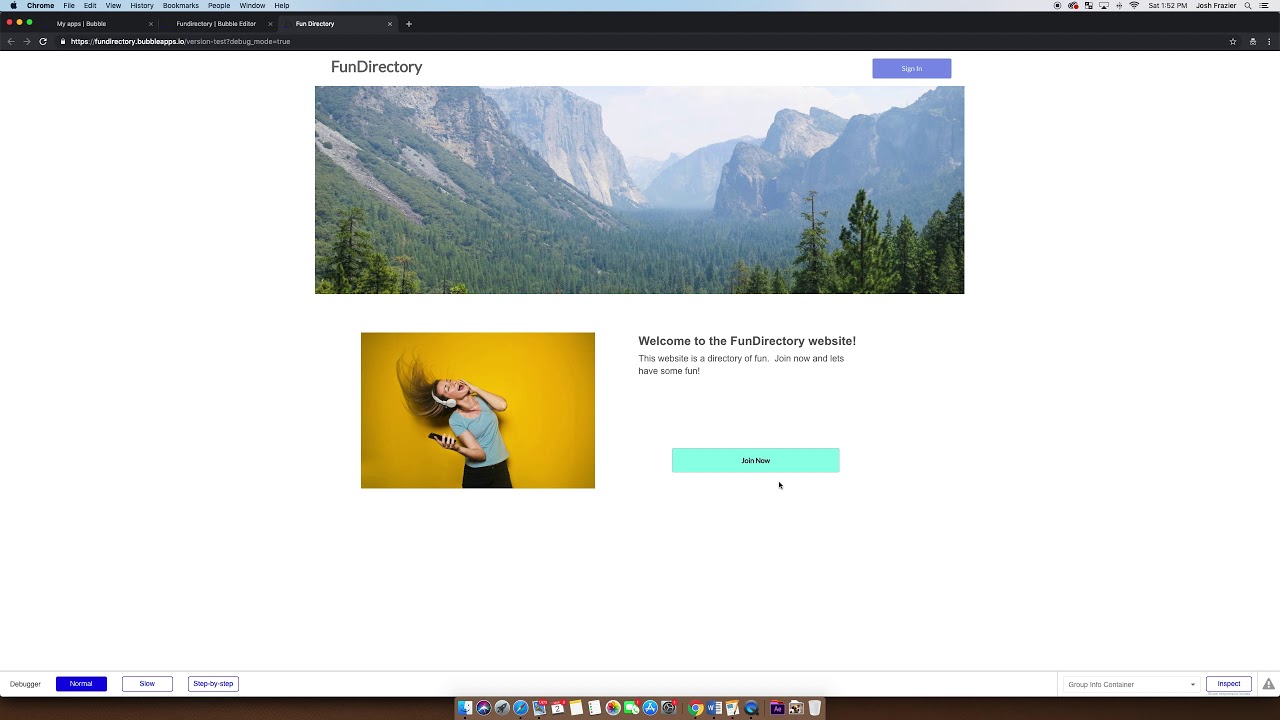The image caption reads "Fun Directory" and features a view of the Rocky Mountains under a light grayish-blue sky. Descending from the mountains, a dense forest of green and evergreen trees can be seen. The phrase "Fun Directory" appears prominently, with a blue "Sign In" banner on the right against a white background.

Below this mountain scene, there's a square picture with a gold background. The image depicts a girl with long, blondish-brown hair tossed in the air. She is wearing white headphones, a short-sleeve gray top, and black pants or shorts that cut off at the thighs. Her left hand rests on her cheek, and she appears to be singing, with an unidentified object in her right hand.

To the right of this second picture, text reads: "Welcome to the Fun Directory website. This website is a directory of fun. Join now, and let's have some fun." Directly below this text is a turquoise banner with "Join Now" inscribed on it.

Above the images and text, there is a black banner displaying a series of menu options such as "Chrome File Edit, View History, Bookmarks, People, Windows, Help," alongside a search bar that seems to contain the search query "Fun Directory." 

The web address is partially visible, showing "HTTPS, Fun Directory..." but is difficult to read completely due to small text size. On the far right, the name "Josh Frazier" is displayed with a series of icons to its left, and the time "Saturday, 1.52 p.m." Below this, there is a black strip with another blue banner above it that is partially readable, showing "Debugger" and another section with "Slow" and "Step-by-Step." Various small icons are located at the bottom, with text on the right reading "Group Into Container" and "Inspect," albeit faintly.